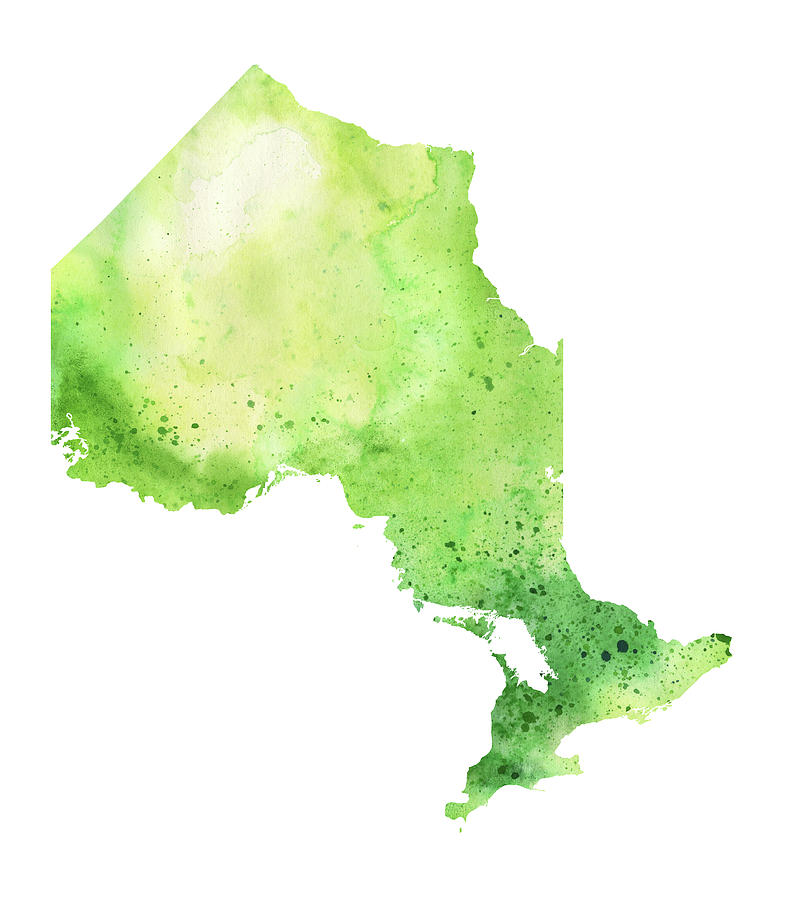The image displays an interpretive artwork or possibly an aerial view resembling the outline of a landmass against a pristine white background. Dominating the center of the image is an oblong, irregularly shaped figure predominantly colored in various shades of green—ranging from dark green to a very light, almost yellowish green—accentuated with black specks. This shape, devoid of any text or distinct features, evokes the appearance of a country, peninsula, or land map. The artistic rendering lacks clarity in its definition, resembling a blend of abstract shapes and colors with a somewhat distinguishable yet enigmatic form.